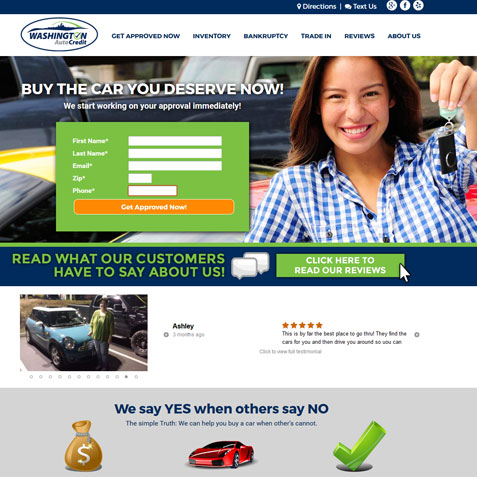The image features a comprehensive interface for Washington Auto Credit, providing various interactive elements for potential car buyers. At the top, there are blue navigation bars with options like "Directions," "Text Us," "Google," and "Facebook." Below, prominently displayed, is a circular logo for Washington Auto Credit, accompanied by a call to action, "Get Approved Now." Nearby, there are tabs labeled "Inventory," "Bankruptcy," "Trade-In," "Reviews," and "Buy This."

In the center, you'll find a bold statement: "Buy the car you deserve now!" followed by the assurance, "We start working on your approval immediately." A green square below includes form fields for "First Name," "Last Name," "Email," "Zip Code," and "Phone Number," all accompanied by an asterisk indicating mandatory fields. This section is completed with a prominent red button labeled "Get Approved Now."

Underneath, a large blue bar with green text invites users to "Read what our customers have to say about us," featuring two comment bubbles and a clickable link to customer reviews. Beside this text is an image of a smiling woman with short hair, holding a phone or key fob.

A testimonial section features a picture of a customer named Ashley from three months ago, standing next to a mint blue Mini Cooper while wearing a green sweater. Her review highlights the excellent service, stating, "This is by far the best place to go to find the cars for you, and then drive you around so you can have something." A call to action prompts users to "Click to see the full review."

Lastly, a gray square at the bottom reinforces Washington Auto Credit's customer commitment: "We say yes when others say no," with the promise, "We can help you buy a car when others can't." This section includes icons of a bag of money, a sports car, and a green check mark, emphasizing financial assistance, luxury, and approval.